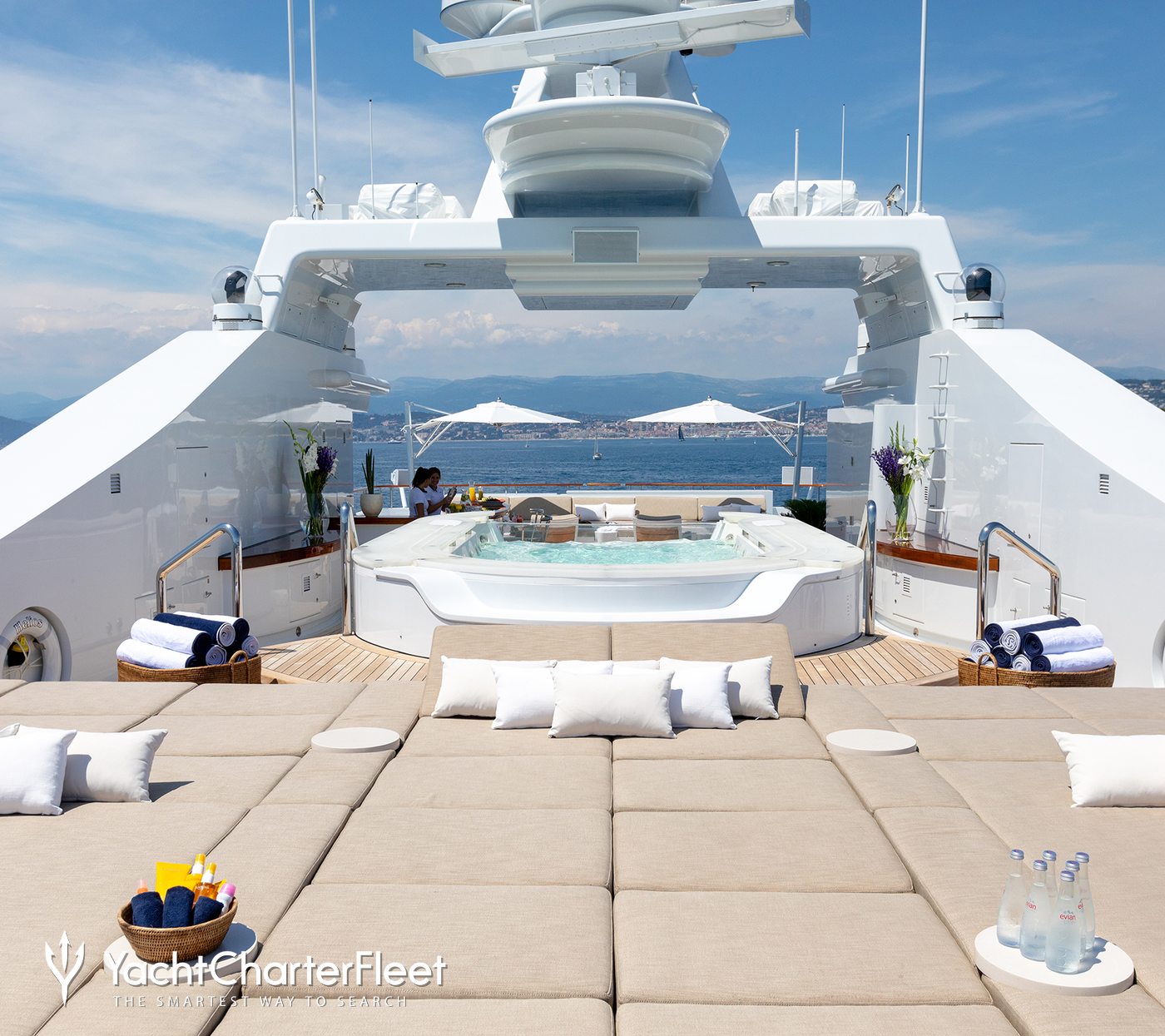The image showcases the luxurious deck of a pristine, white yacht, viewed from the mid-section towards the front (bow). The deck is adorned with beige and white cushions and pillows artfully arranged for comfort. A stylish picnic setup is present, featuring a serving tray with fancy bottled water, napkins, and a basket, all suggesting a sophisticated charter experience. Positioned at the front are two individuals in crisp white polos, possibly staff members, standing by a desk, hinting at the yacht's exclusive service.

In the foreground, the wooden deck extends elegantly, populated with potted plants with blooming flowers and baskets, possibly containing towels or other amenities. Highlights include a clear swimming pool towards the back (stern) and a luxurious hot tub at the bow, indicating the yacht's opulent features. Technological equipment, possibly a radar, is subtly visible above, adding to the vessel's advanced and high-end appeal. The open, unobstructed view to the ocean reinforces the yacht's exclusiveness and the serene luxury it offers.